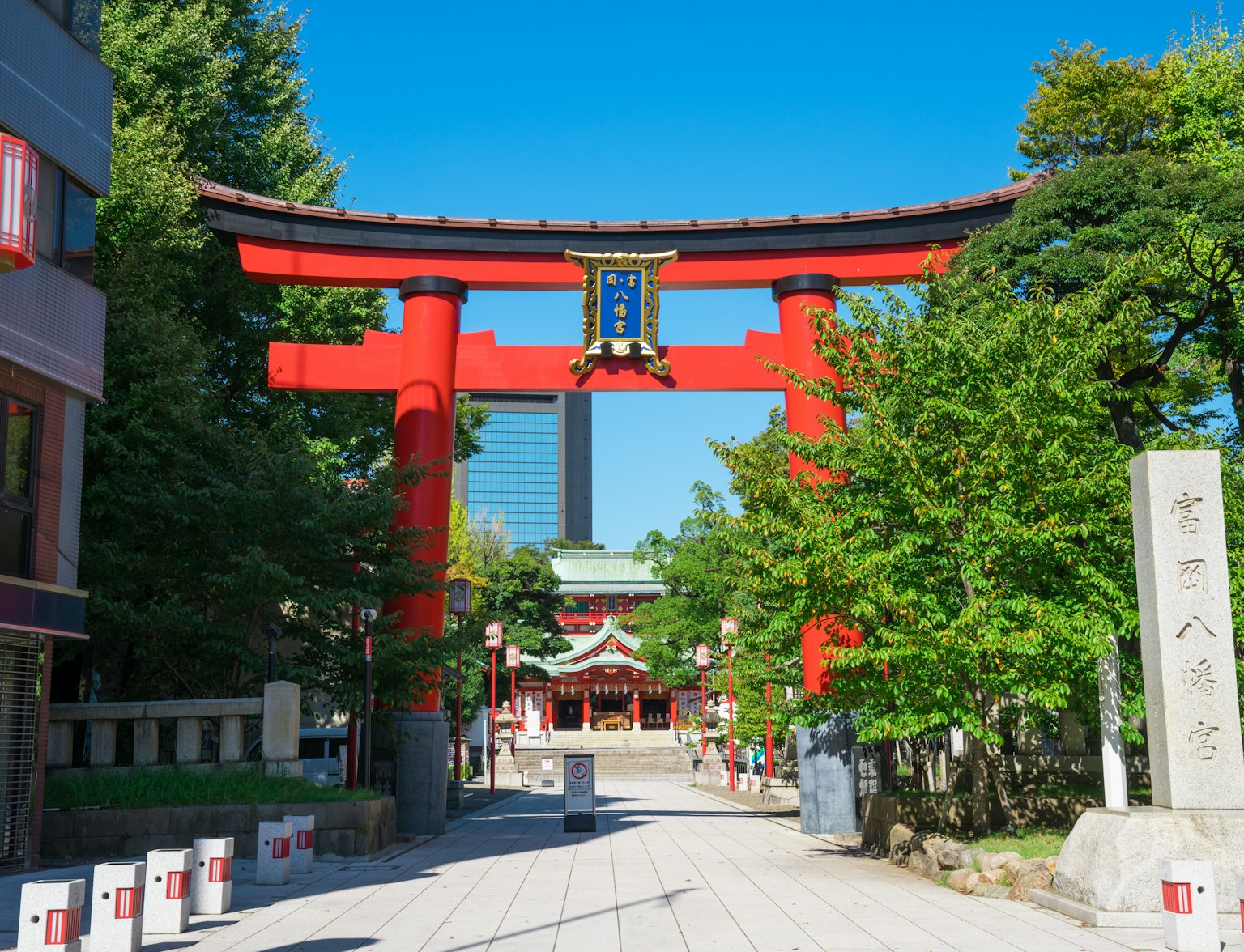The photograph captures a serene walkway leading up to an ornate red and black torii gate, emblematic of Chinese or Japanese architecture, likely marking the entrance to a temple. The gate features a striking blue plaque with gold Asian characters framed in gold, suggesting cultural and spiritual significance. Beyond the gate lies a small temple with red walls, detailed accents, and a light green roof. The scene blends traditional and modern elements: the stone pathway and bright green trees contrast with streetlights dotting the sidewalk and a dark concrete building to the left. In the background, a skyscraper looms, emphasizing the juxtaposition of ancient heritage and contemporary cityscape.